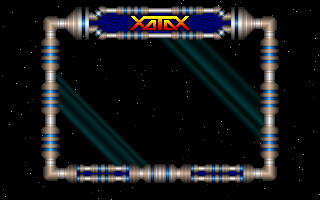This is a small, color photograph of a digitally generated image, likely a screen capture from a video game, featuring a predominantly black background sprinkled with tiny white specks resembling stars. The central focus is a rectangular structure that resembles cylindrical metal pipes segmented with horizontal bands. These bands are primarily beige and blue and curl around the outer edges of the structure. 

At the top of the structure is a prominent blue rectangular sign with the text "XATAX" written in capital letters; this text is gradient colored with yellow at the top and red at the bottom. The sign is flanked by large "X" symbols on either side of the text, which is somewhat difficult to decipher. 

Within the interior of this rectangular structure, we see horizontal green lines running from the upper left to the lower right at the top and bottom. Additional blue, fluorescent horizontal lines are present along the split areas of the structure, further segmented at the edges. The pipes or bands have a detailed texture, giving the structure a dimensional quality that enhances the digital aesthetic of the image.